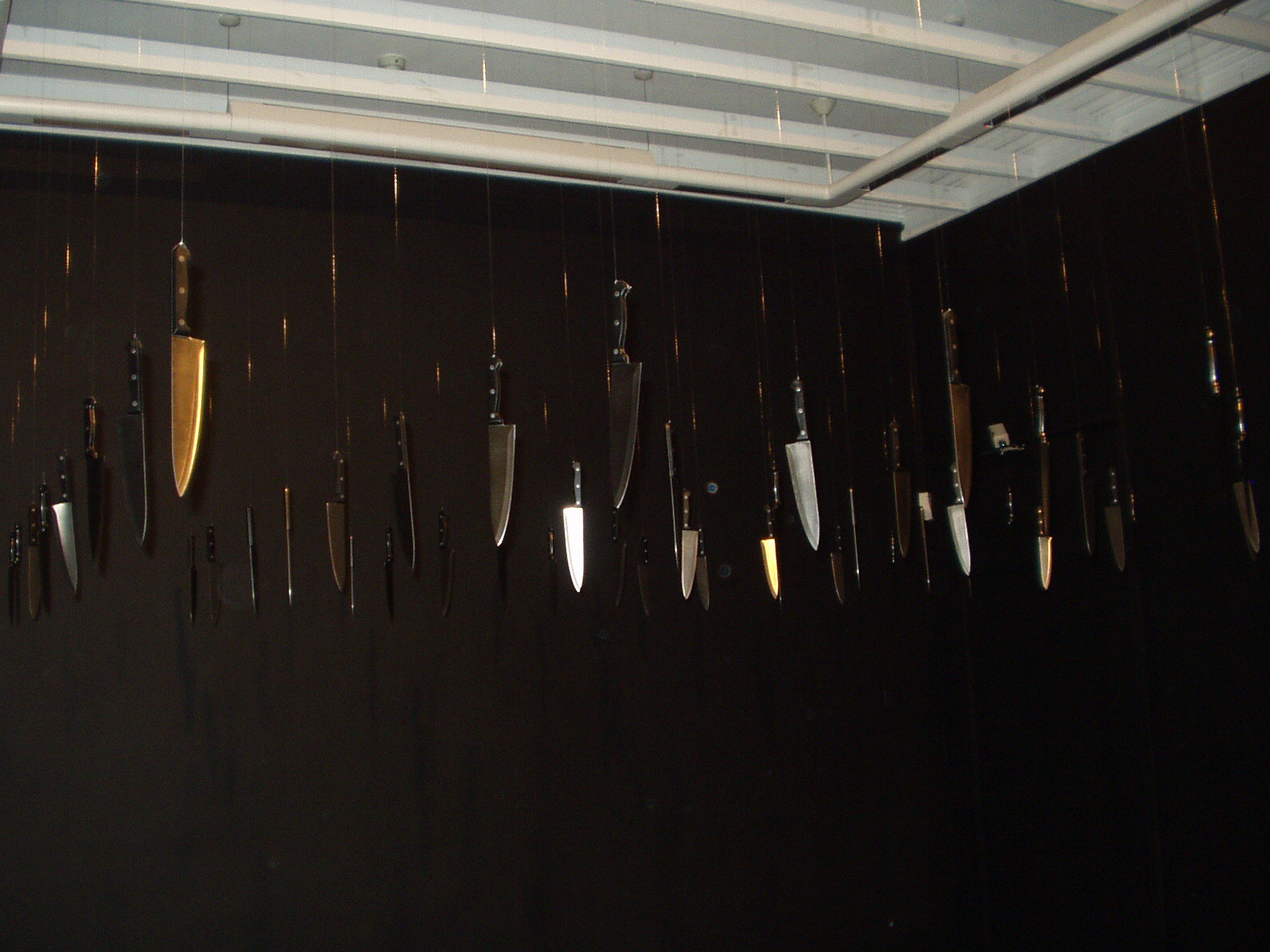The image showcases an eerie room where approximately 40 to 50 large butcher knives are suspended from the white ceiling by clear fishing lines. Each knife hangs handle-up, blade-down, with their sharp edges gleaming under the light. The knives are primarily uniform in size, featuring either silver or gold blades, with black or brown handles. The upper portion of the image reveals a white ceiling accented with some piping, while the lower two-thirds of the image is enveloped in darkness, suggestive of black screens covering the walls. This backdrop enhances the sinister atmosphere, as the multitude of gleaming knives dominate the composition, their reflections creating a haunting visual effect.